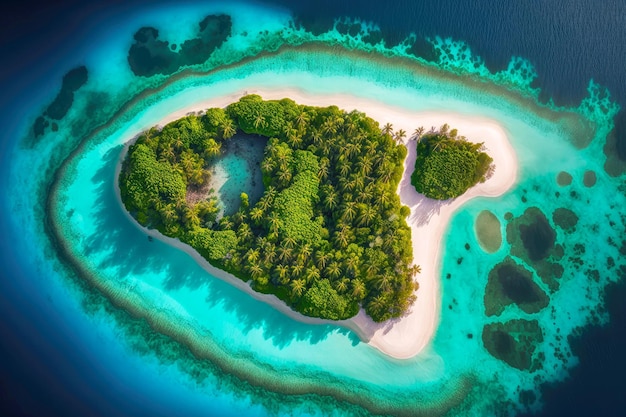This aerial photograph captures a strikingly picturesque, tiny oval-shaped island that resembles a capital "A" formation. Dominated by a dense forest of trees and shrubs, the island features a distinct opening at its peak. Surrounding the lush greenery is a pristine white sandy beach that extends outward, especially prominent on the right-hand side, splitting into two sections. The immediate waters around the island display a breathtaking gradient, starting with very light turquoise blue—likely due to the shallowness and reflection of the sandy bottom—transitioning to a richer, medium aqua, and finally deepening into a dark, intense blue as the ocean depth increases. The water in proximity to the island appears slightly churned and frothy, mixing with the surrounding sand and giving the appearance of sea foam or lighter green patches amid the vibrant array of blues. This untouched gem in the middle of the ocean suggests a sense of serene isolation and natural beauty.